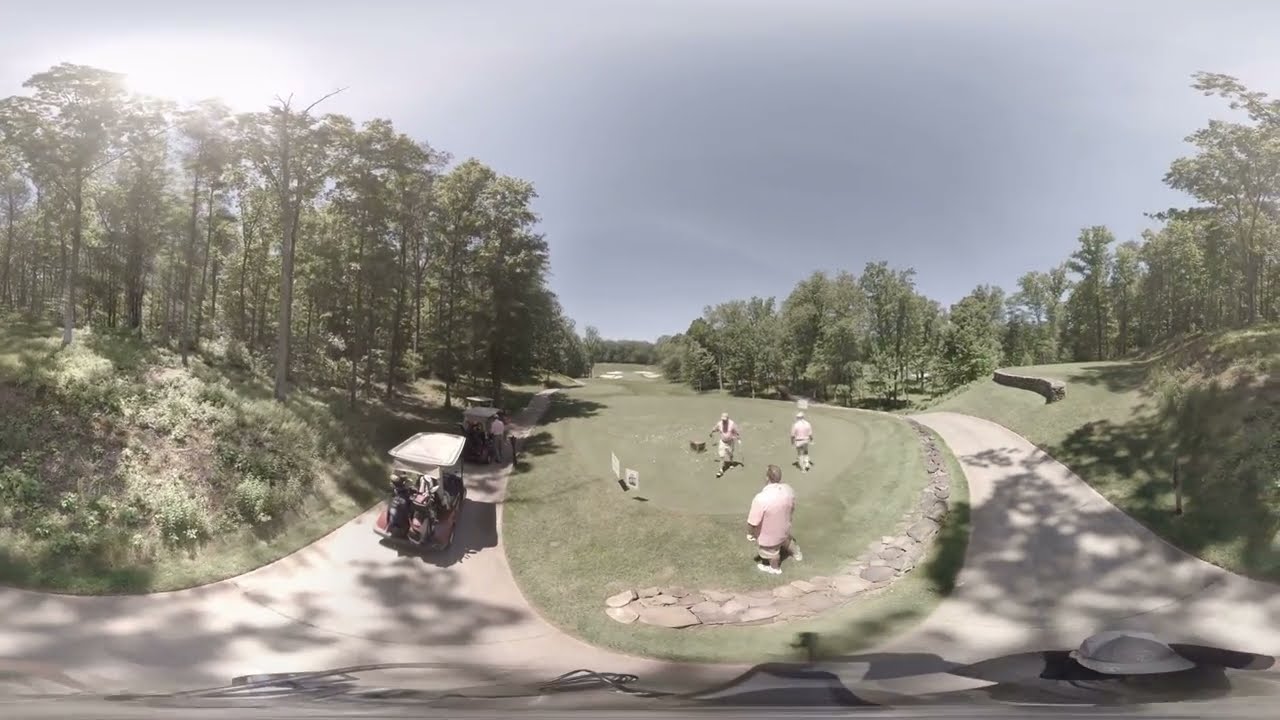In this vibrant and sunlit golf course scene, three gentlemen are preparing to tee off on a lush, green tee box. They are all dressed in light-colored clothing, comprising white collared shirts, shorts, and caps. The central figure, clad in a white short-sleeved shirt and khaki pants, is walking up to the tee box to set up his shot. To the left of the players are two golf carts parked on a concrete path. The path separates and encircles the well-manicured lawn, adorned with strategically positioned cobblestones. Framing the picturesque scene are verdant trees under a bright, cloudless blue sky, casting minimal shadows owing to the high sun. In the distance, approximately 400 yards away, sand traps dot the fairway, providing potential hazards for their game. Additionally, a portion of the course to the right is demarcated by a stone wall, hinting at another hole adjacent to the current one. The serene beauty of the course, combined with meticulous details, paints a perfect day for a round of golf.